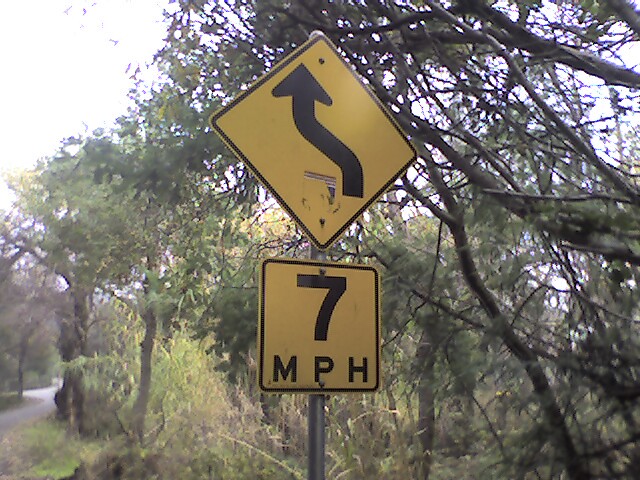In this photograph, the focal point is a pair of traffic signs mounted centrally on a galvanized metal pole. The top sign is diamond-shaped and yellow with a black border, featuring an arrow directing both left and straight ahead. Directly below, a rectangular white sign indicates a speed limit of 7 MPH. The background is somewhat blurry, showcasing an overexposed sky in the top left corner. A collection of scrubby trees fills the scenery, and a narrow strip of road is visible on the extreme left edge of the image.